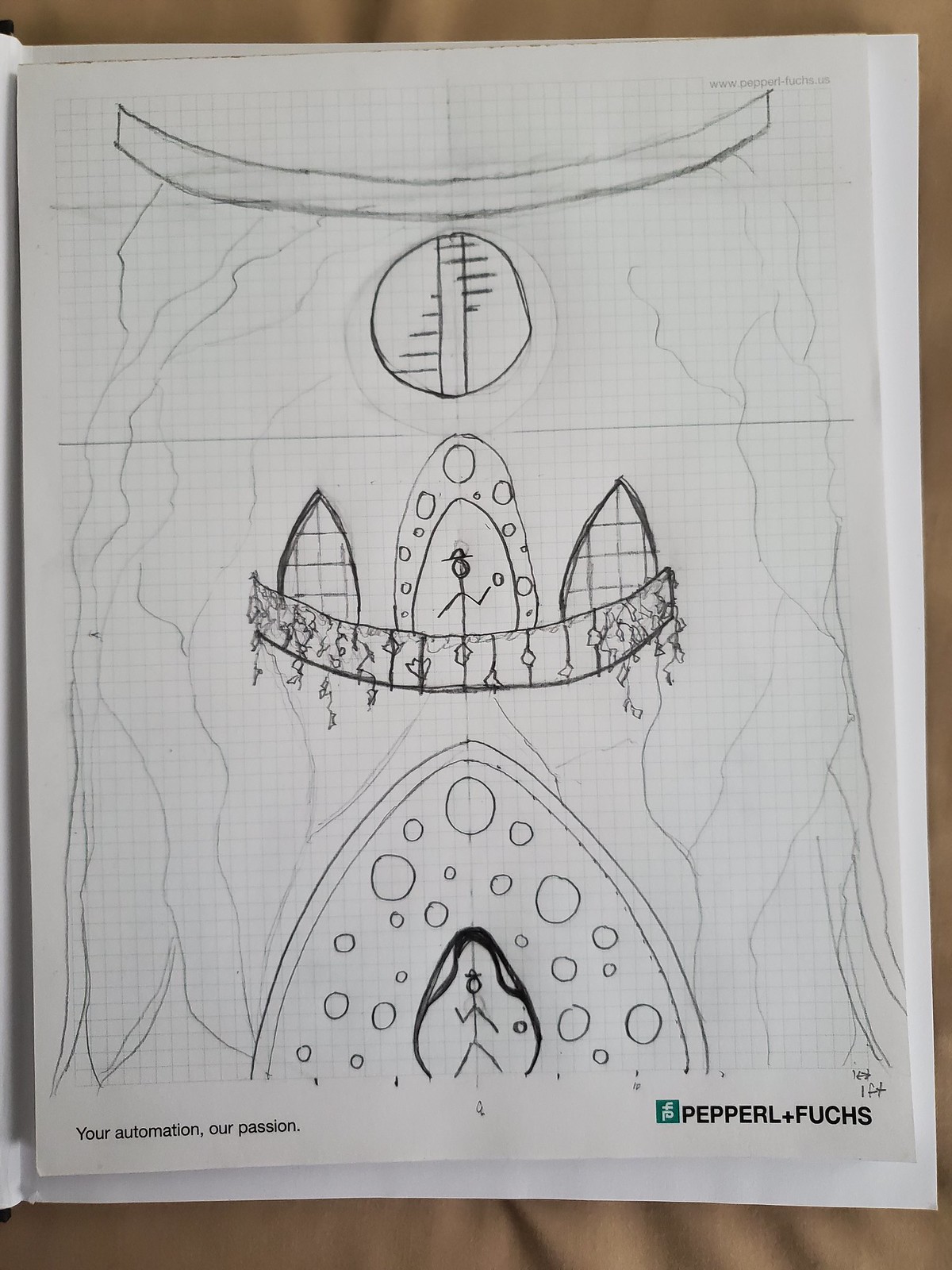In this image, a light brown cloth serves as the backdrop for a piece of light gray paper, which features a detailed pencil drawing. The central subject of the drawing is a large building with an architectural design resembling a cave entrance at the bottom, tapering upwards to form an upside-down V shape. Inside this V shape are small circles, adding texture or detail. Above this structure, another smaller upside-down V contains a stick figure. Below this, the text "Pepper and Fuchs" is written in black, accompanied by a green insignia, and the phrase "Your animation, our passion" is also present. 

Further details of the building include a balcony, from which various small objects are hanging. Two large windows sit prominently on the facade, and another doorway below contains another stick figure. Dominating the upper portion of the drawing is a large circle, inside which a spiral staircase is depicted, suggesting an intricate interior space.